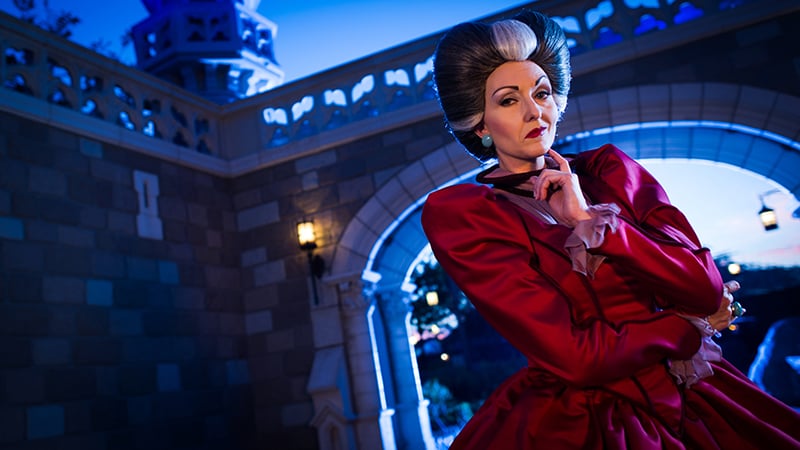In the image, a person is dressed in an elaborate costume as the Wicked Stepmother, Lady Tremaine, from Cinderella. She wears a wig styled in a distinctive, bulbous pattern with mostly brown hair accented by three gray spots. Her makeup is done in an exaggerated fashion, featuring arched eyebrows, noticeable rouge, and dark lipstick. Her ears are adorned with circular light blue earrings. She dons a deep red, Victorian-style dress with frilled purple lace around the wrists, completing her striking appearance.

She stands in an ornate castle setting, under an archway shaded by wrought iron lanterns. One lantern is positioned in a sconce while another hangs from a metal fixture; additional lanterns are faintly visible in the background. Nearby, there is a small window embedded in a castle wall, and a cement railing is seen above. In the far corner, a castle tower adds a majestic touch to the scene. Her dramatic expression and detailed costume vividly bring the character to life, making her resemblance to the Wicked Stepmother unmistakable.